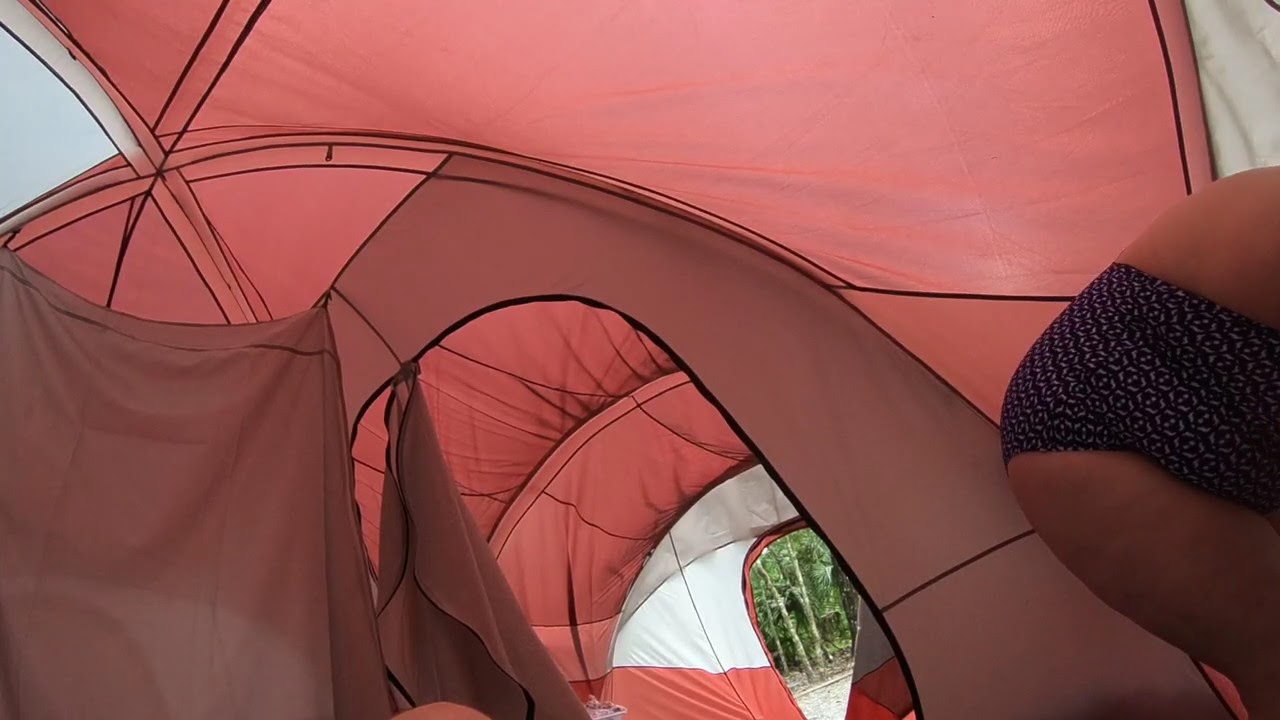The image captures the interior of a parachute fabric-like tent structure with a tunnel-like design. This horizontally aligned rectangular image highlights the tent's vibrant red and white sections, divided by thin black bands. The top part of the tent is predominantly red, contrasting slightly with the red shades in the middle and bottom sections. On the right side of the image, a woman is bent over, her upper back bare while the rest of her body is clad in a swimsuit with a white pattern. The visible part of her body includes her midsection and the right side of her left thigh. Toward the end of the structure, a hole reveals an outdoor scene with green leafy trees and a dirt pavement, with some gravel visible on the ground. This opening suggests a crawl space leading in and out of the tent.